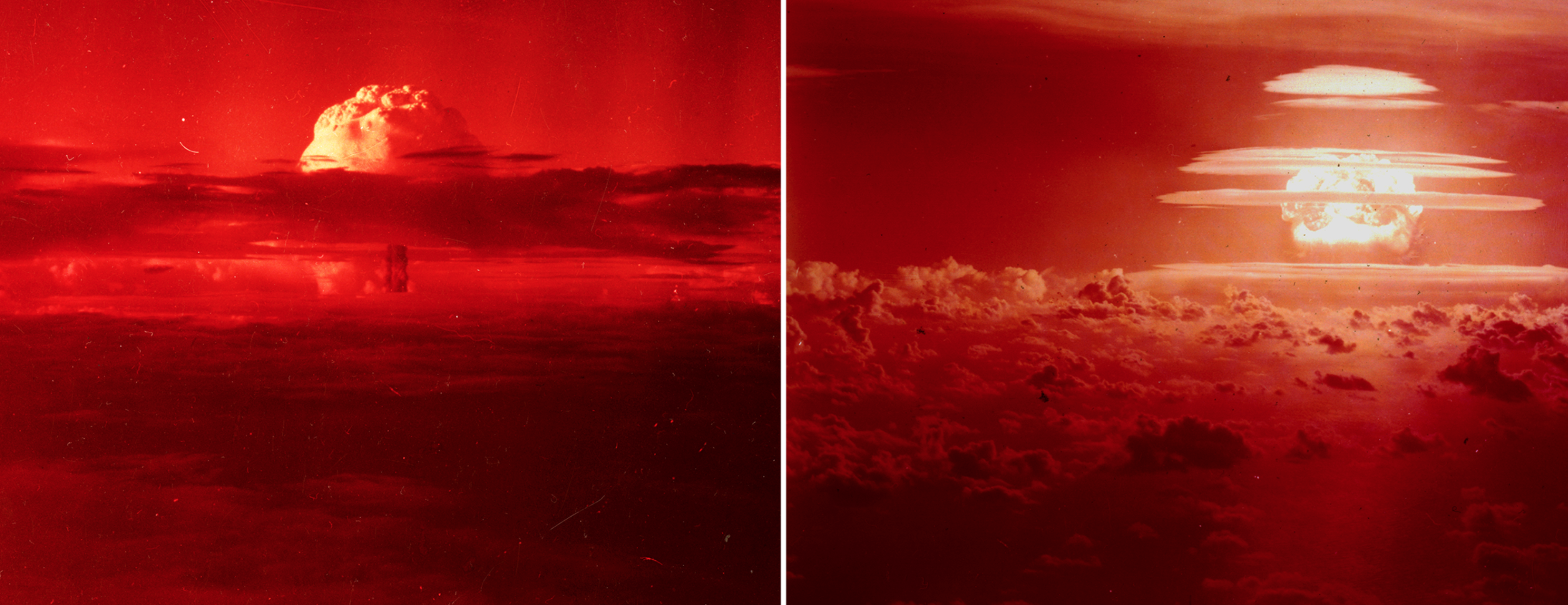The image is actually a collage of two pictures, each depicting a striking scene from above the clouds that could be a sunrise or sunset. The left picture showcases dark, cloudy bottoms with strips of lightness and deeper layers of clouds. Above these layers, a large white cloud resembles a scoop of ice cream, set against a backdrop of deep, fiery red, causing the whole scene to bathe in a mysterious reddish hue. The sky transitions from dark brown and white clouds to a radiant deep red, accentuated by striking light and shadow contrasts.

The right picture features a cluster of rolling, lumpy red clouds at the bottom, ascending into a lighter yellow and then a very bright region that resembles the setting sun. This bright area is accompanied by dark cloud strips and a cloud dome overarching it. The sky in this frame evolves from a red base to illuminated golden-yellow hues, giving the impression of an otherworldly, fiery event. The entire scene has a magnificent deep red theme, with complex cloud formations and grand contrasts of light. They evoke a sense of witnessing either a natural phenomenon like a dramatic sunset or an extraordinary celestial event.

In summary, the two pictures vividly capture a breathtaking panorama, blending dark, cloud-laden skies with radiant fiery tones, giving an impression of both a peaceful celestial twilight and an explosive, almost mushroom-cloud-like spectacle. The deep red and golden colors dominating both images paint a surreal and captivating vision.